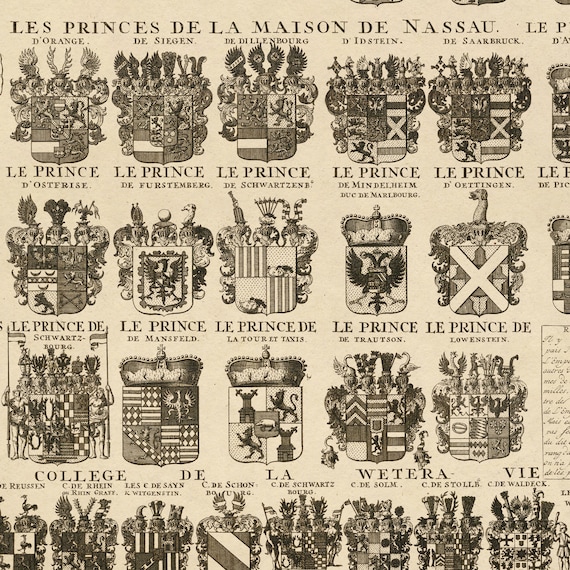This square image appears to be an aged, sepia-toned poster featuring historical coats of arms and crests of various princes, potentially of European origin, likely from France given the French text. The background is a light tan, evoking an antique feel. The poster is organized into four rows of side-by-side shields, with five shields in the first three rows and eight in the bottom row, where the shields are cut off at the bottom. At the top, in all capital letters, it reads "LES PRINCES DE LA MAISON DE NASSAU." Each crest is intricately illustrated in black and white, depicting various symbols such as birds, wings, lions, and crowns. Each shield is labeled with titles such as "d'Orange," "de Seguin," "de Dillenbourg," "d'Edstein," and "de Saarbrück," with similar labels in the other rows. There is a partial cursive inscription near the mid-right corner of the poster, enhancing its historical essence.